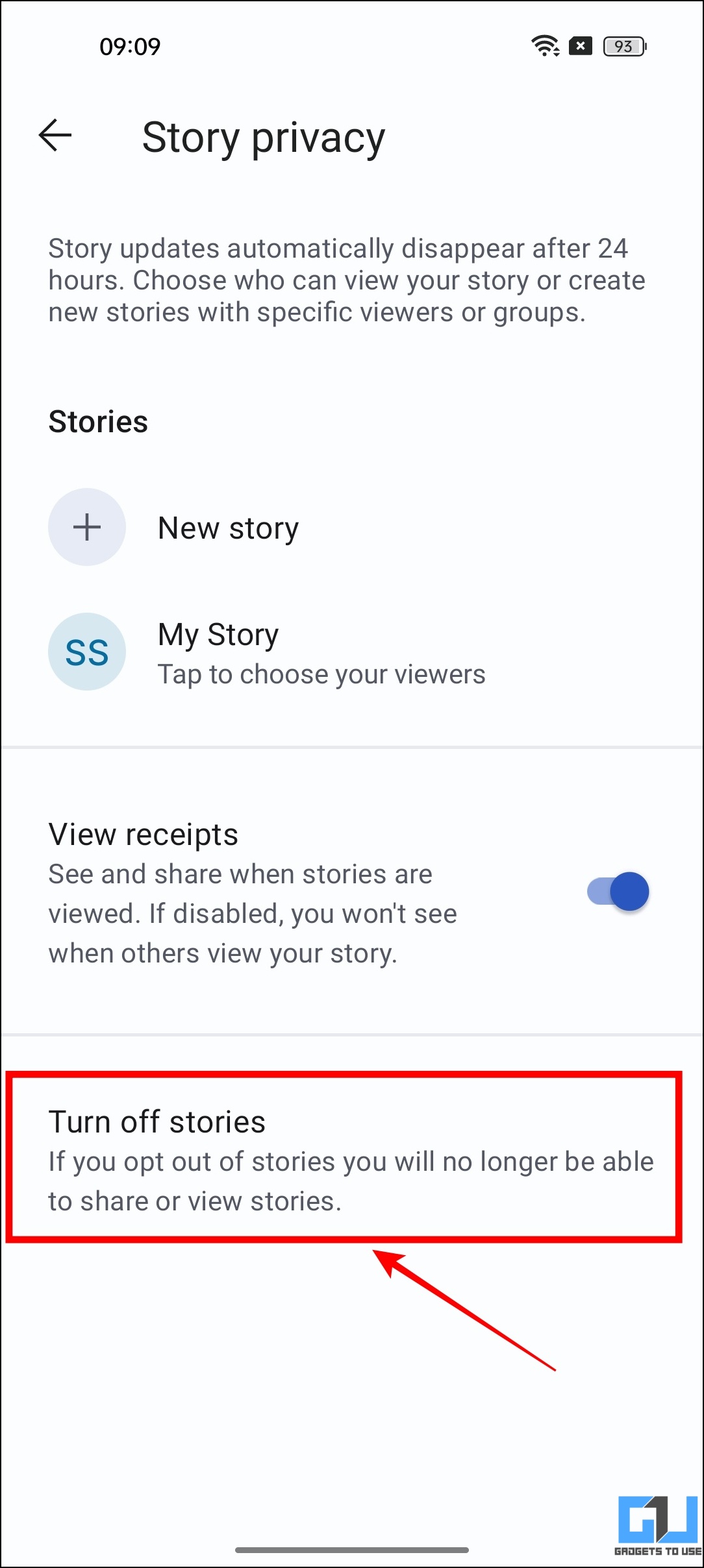The image has a black border surrounding a white background. At the top of the image, the display shows "9:09" with a full Wi-Fi icon and 93% battery, indicating no SIM card is inserted. Beneath this are interface elements including a left-pointing arrow labeled "Story Privacy".

The screen also contains text in gray: "Story updates automatically disappear after 24 hours. Choose who can view your story or create new stories with specific viewers or groups." Further down, it shows a "Story" subsection with a plus sign labeled "New Story" followed by "SS, My Story." 

Text prompts users to "Tap to choose your viewers" and informs about "View Receipts: See and share when stories are viewed." A blue slider indicates the view receipts feature is enabled.

Additionally, there's a red square with a red arrow pointing to it, highlighting text in black: "Turn off stories: You can opt out of stories. You will no longer be able to share or view stories." At the bottom center, there's a small black line.

The image also contains what appears to be a screenshot with some text that looks like "G and U" or "G1 backwards L" in light and dark blue with something black underneath, which might say "gadgets to win." The exact text is unclear.